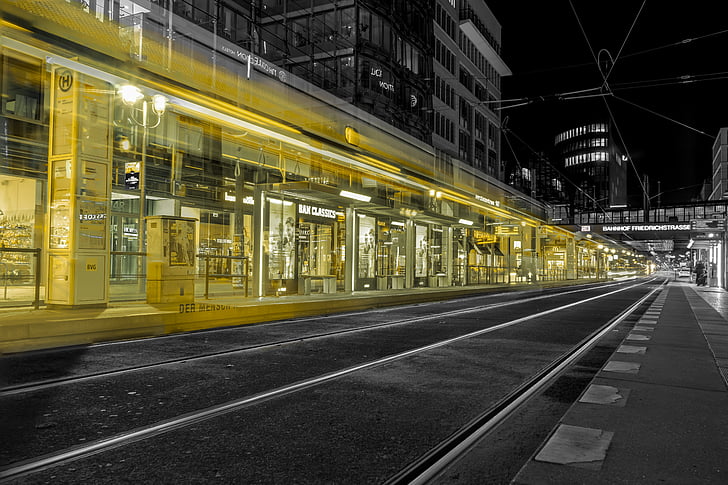This wide-angled night-time photograph captures a long city street adorned with tracks for a cable car, trolley, or light rail system. The image is predominantly black and white, with a vivid streak of yellow highlighting the ground floors of storefronts on the left side. The street, starting diagonally from the bottom left corner and extending to the center-right, features tall buildings with many windows softly lit in the background, and a web of cables crossing the dark night sky above. The yellow coloration, possibly a digital after-effect or a motion blur, suggests an active waiting area or station. A pedestrian bridge spans further down the street, while one of the storefronts, labeled "B&M Classics," stands out among numerous glass-fronted shops. The overall scene conveys an urban, tranquil atmosphere lit by scattered lights amidst the enveloping darkness.